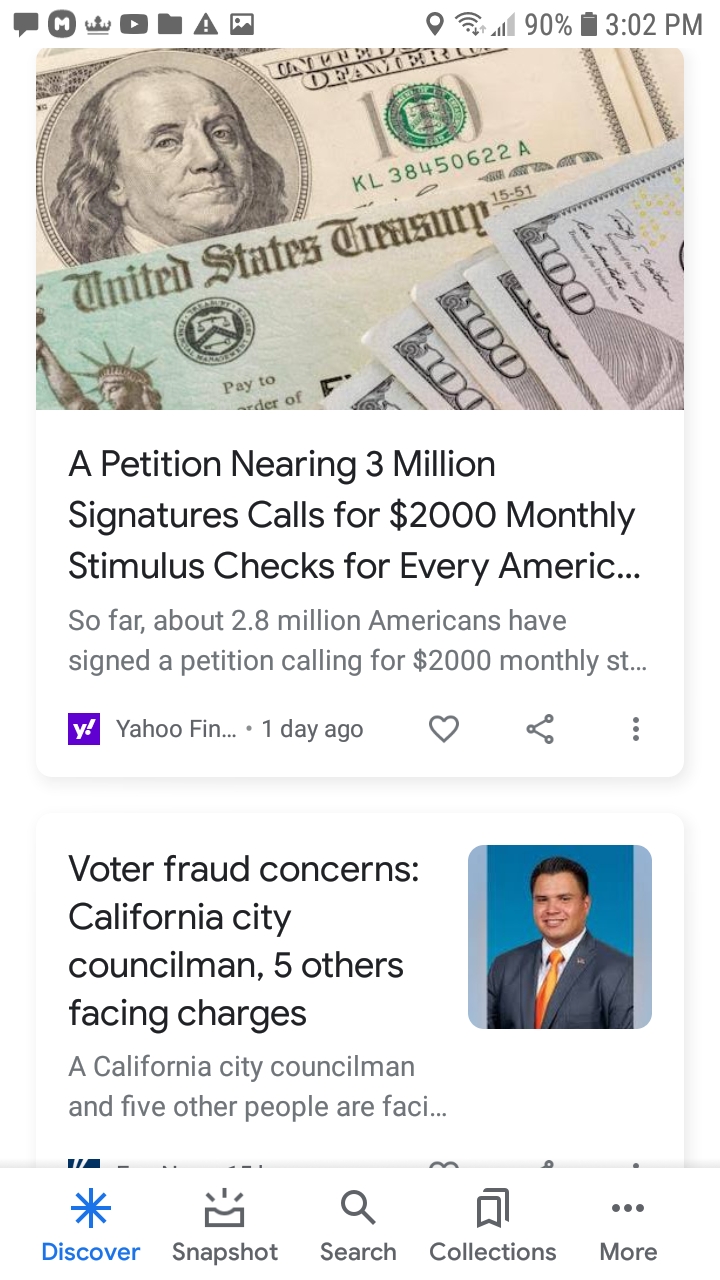This image captured from an iPhone shows the screen at 3:02 p.m. with 90% battery life and a strong connection signal. The screen displays multiple app icons on the left side, some in solid black. The main content shows a headline from Yahoo Finance, dated one day ago, that reads, "A petition nearly 3 million signatures calls for $2,000 monthly stimulus checks for every American." Below the headline, the article mentions that about 2.8 million Americans have signed the petition. Visible on the screen are images of U.S. Treasury bonds and a corner of a $100 bill. Another news snippet highlights concerns about voter fraud involving a California City Councilman and five others facing charges. The image appears to have been captured with another screen overlay beneath it, showing options like "Discover," "Snapshot," "Search," "Collections," and more along the bottom, suggesting some functionality overlap or app interaction.